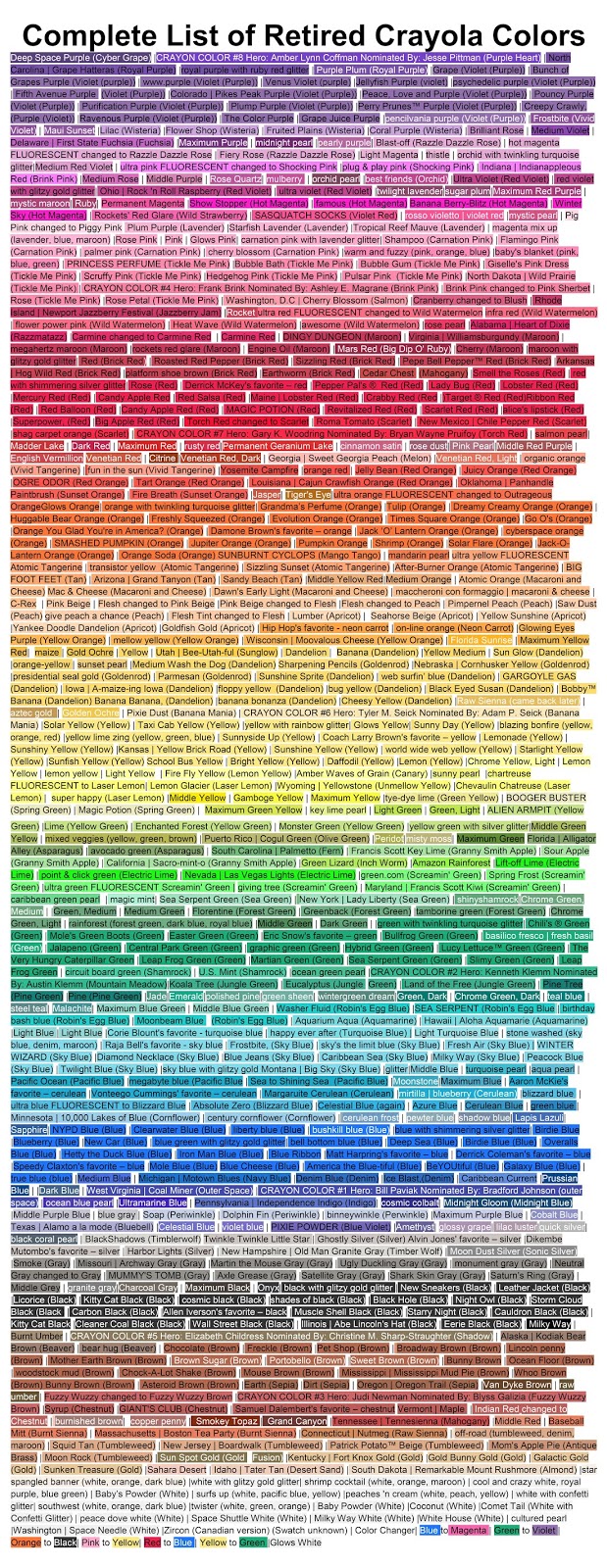The image features a detailed compilation titled "Complete List of Retired Crayola Colors" displayed against a white background. The list comprises an extensive enumeration of color names, highlighted in the respective hues they represent, creating a visually striking rainbow effect. Starting at the top with deep purple shades, the colors transition through various tones of purple and lavender, moving into pinks and magentas, then light reds to deep reds. This gradient continues into oranges, yellows, various greens, from dark to light, transitioning into blues—from turquoise and light blue to deep navy. The progression leads into grays and blacks, finally culminating in rows of colors at the bottom that range from whites to marine hues. Despite the small and dense lettering, the myriad of colors artistically arranged from top to bottom vividly showcases the breadth of Crayola's retired palette. This artistic representation captures the nostalgic spectrum of colors that have been discontinued over the years.